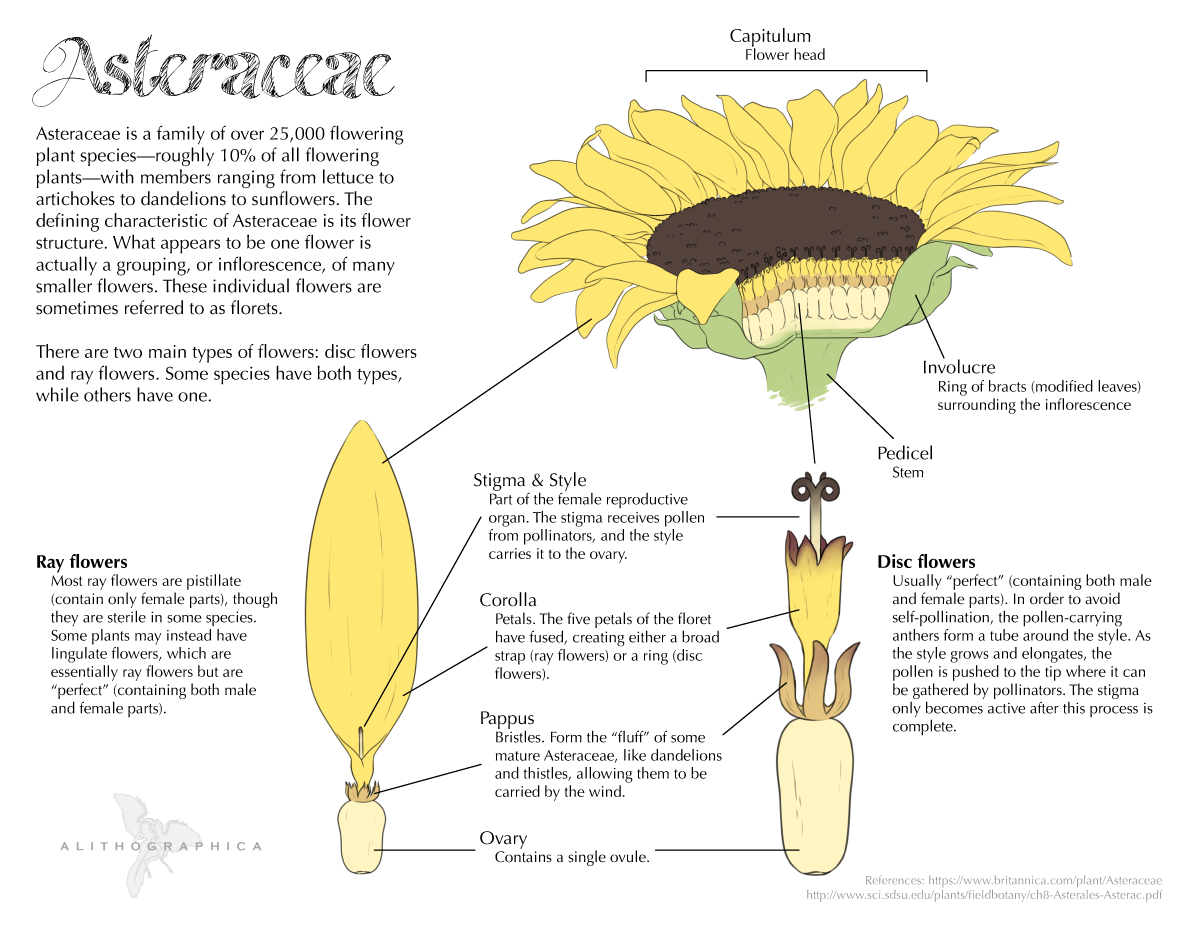This image is a detailed botanical diagram from a book titled "Alithografica,” depicting the Asteraceae family, which comprises over 25,000 flowering plant species, accounting for roughly 10% of all flowering plants. Examples in this family include lettuce, artichokes, dandelions, and sunflowers. The diagram features an open and a closed sunflower, illustrating the unique structural characteristics of Asteraceae flowers. It emphasizes that what appears to be a single flower is actually an inflorescence composed of many small flowers, known as florets. 

The diagram points out and labels parts of the flower, such as the flower head, involucre, pedicel, disc flowers, stigma and style, corolla, pappus, and ovary, with a horizontal layout that provides a comprehensive overview of each part's function. The color scheme consists of yellows, browns, light browns, and greens, enhancing the detailed explanation of this family's floral structure. The black font text offers a succinct description below the flower name and a more extensive explanation of the different parts and characteristics of the Asteraceae flowers.